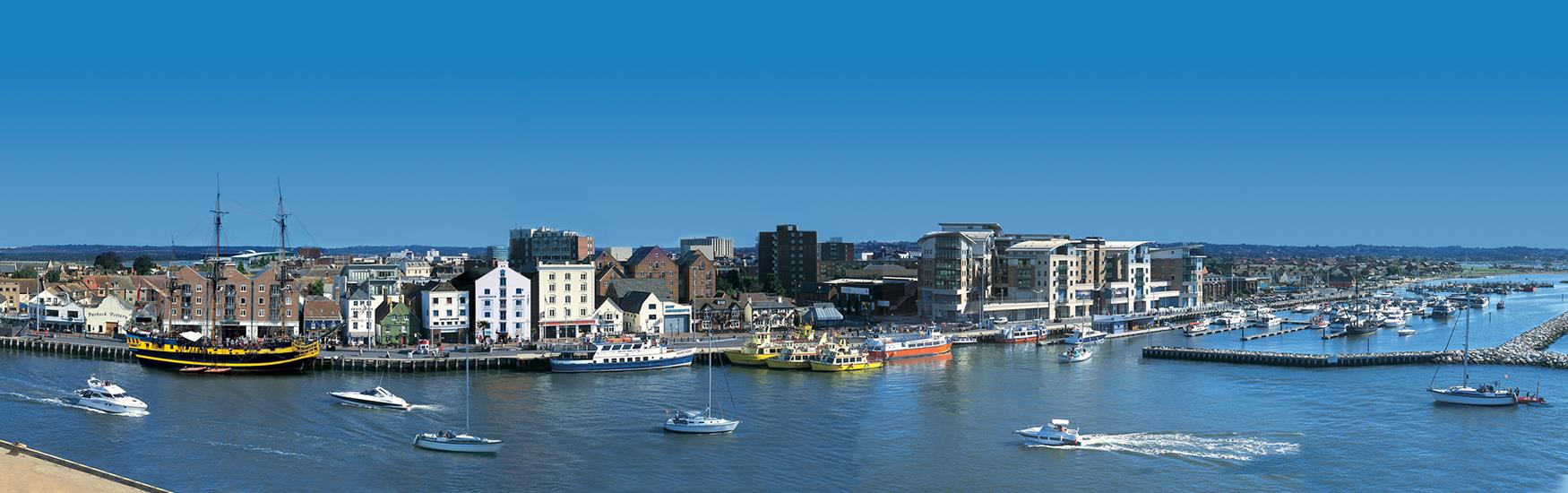The image depicts a panoramic, wide-angle view of a bustling cityscape adjacent to a clear blue waterfront under an all-blue sky. The clear water, reflecting the similarly blue sky, is dotted with several boats. In the foreground, there are five to six active boats leaving white trails, including speedboats and sailboats without their sails up. Midway in the water, you can spot small yellow boats and a large black and yellow barge or ferry. To the left, the shoreline is crowded, likely featuring a marina, with some visible cranes behind the buildings. The buildings along the water vary in color, transitioning from brownish brick structures on the left, to white in the center, and beige or cream towards the right. Mid-rise buildings, both residential and commercial, form the cityscape, with occasional darker brown buildings adding to the visual variety. In the background, hills or mountains provide a scenic backdrop to the striking waterfront city.